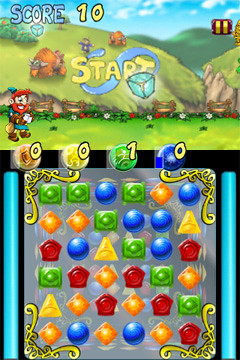The image depicts a mobile video game screen in portrait mode. The game appears to be a blend of Tetris and Bejeweled, featuring a puzzle play area at the bottom where players connect matching jewels and shapes to score points. The jewels are in various bright colors, such as yellow diamonds, blue spheres, green squares, and red shapes resembling wax seals, with numbers in their top right corners indicating the count collected. The top section features a picturesque, cartoon-style hillside scene with cows and a leprechaun-like figure with ginger hair and beard, dressed in a blue skirt and brown shoes, carrying a gold bag. The hillside is adorned with small wooden fences, flowers, and green bushes. Prominently in the middle of the screen, the word "START" is written in large yellow letters over a blue swirl and a jeweled box. On the top left corner, "SCORE" is displayed in blue with the current score of 10 in yellow.